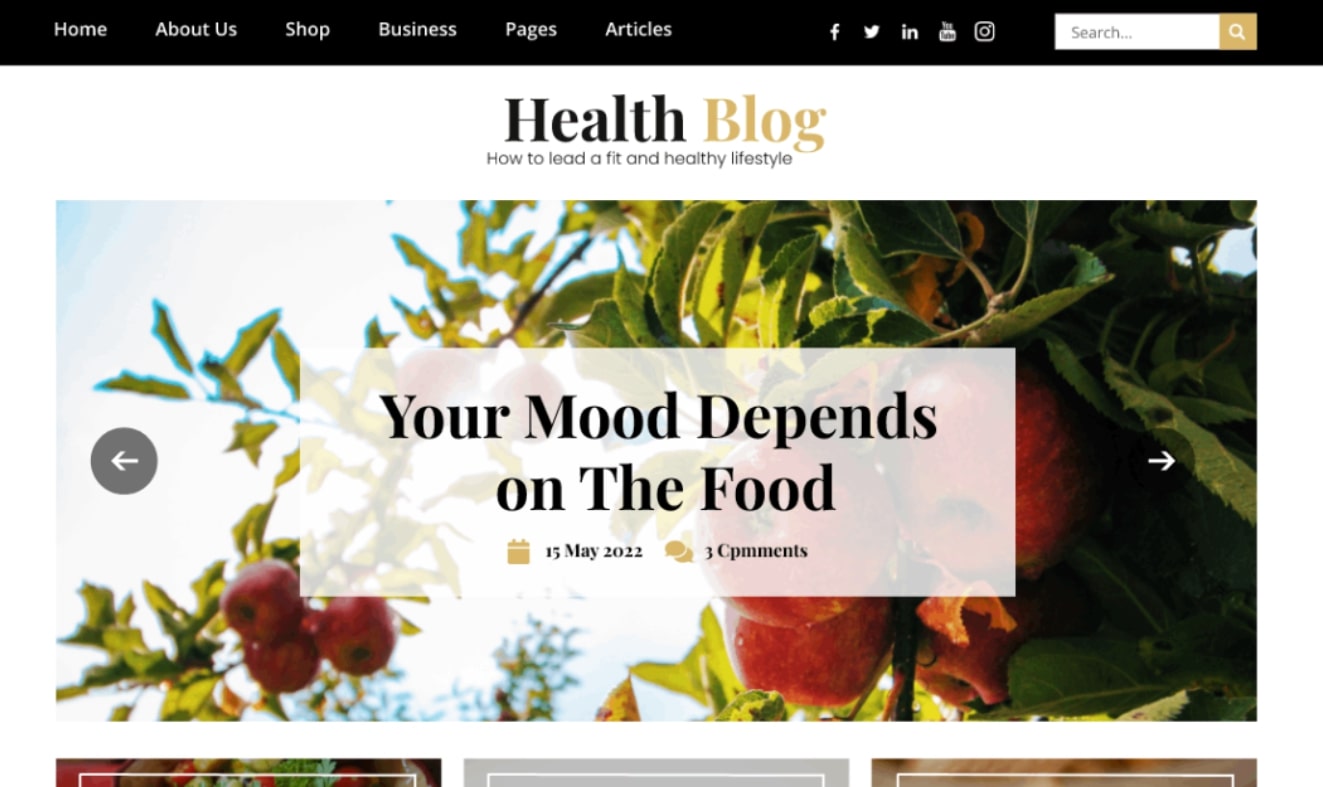This horizontal image appears to be a screenshot from a web page that can be accessed via a smart device or computer. The background primarily utilizes a white color, likely reflecting the default screen color of the user's device. 

At the top of the page, a long black navigation bar spans from left to right. On the upper left-hand side, white text displays clickable options, including "Home," "About Us," "Shop," "Business," "Pages," and "Articles." Moving right, a series of social media icons are available for user interaction. Adjacent to these icons, a white search bar features a tan magnifying glass button.

Centrally, within the white background, bold black text reads "Health Blog," followed by the article title "How to Lead a Fit and Healthy Lifestyle." Below this, there is an outdoor image capturing a serene sky with wispy clouds and sunlight, accompanied by vines bearing fruit.

The bottom part of the image showcases the upper portions of three pictures, slightly cut off. Overlaying this section is a text box that states in black, "Your Mood Depends on the Food," with a calendar icon showing the date "15 May 2022" and a comment icon indicating "Three Comments."